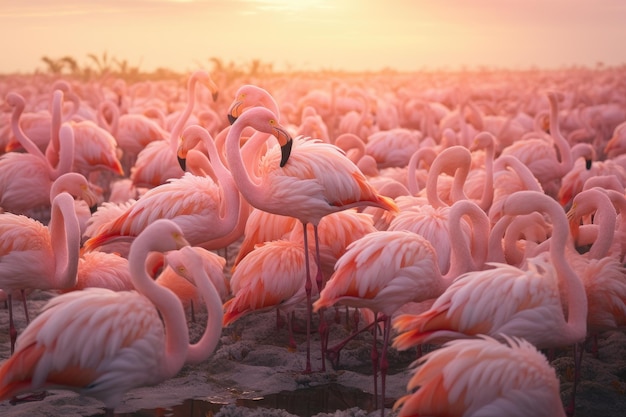The image features a vast congregation of flamingos, numbering in the thousands, assembled in what appears to be a marshland characterized by muddy terrain interspersed with small puddles. The focal point of the image highlights a particularly vivid flamingo, standing upright with its body oriented left while its head turns right. This flamingo, along with others, boasts a pink plumage with darker pink hues accentuating their tail feathers. A striking contrast is provided by their yellow beaks, which transition to black at the front, and matching yellow eyes. The scene extends into a blurred horizon, depicting endless flamingos, some standing, while many are seated, contributing to a sense of depth. Above this immense gathering, a yellow sky, possibly illuminated by a rising or setting sun, casts a warm glow over the landscape. In the distant left, faint outlines of plant life hint at the ecosystem's diversity, while the overall brightness of the day is palpable.